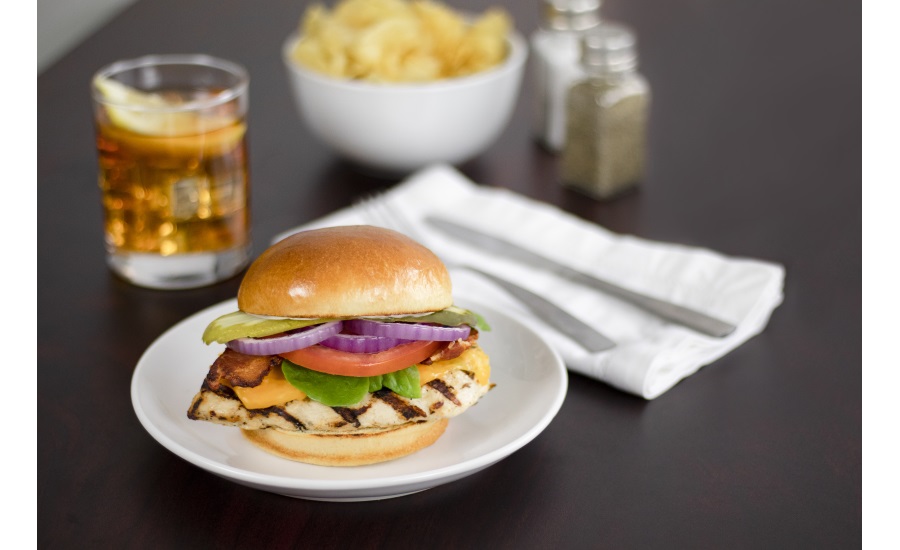This image showcases a meticulously plated grilled chicken sandwich at a restaurant, sitting on a white plate atop a dark mahogany table. The sandwich features a juicy grilled chicken patty nestled in a glossy, buttered brioche bun. Complementing the patty are slices of red onion, tomato, crispy bacon, pickles, and melted cheese, with a hint of mayo. In the background, a blurred glass—likely bourbon or iced tea—with a lemon wedge, sits alongside a neatly folded white napkin with a polished metal fork and butter knife. To the left of the napkin, a white bowl holds either potato chips or macaroni and cheese, while nearby salt and pepper shakers complete the classic table setting.